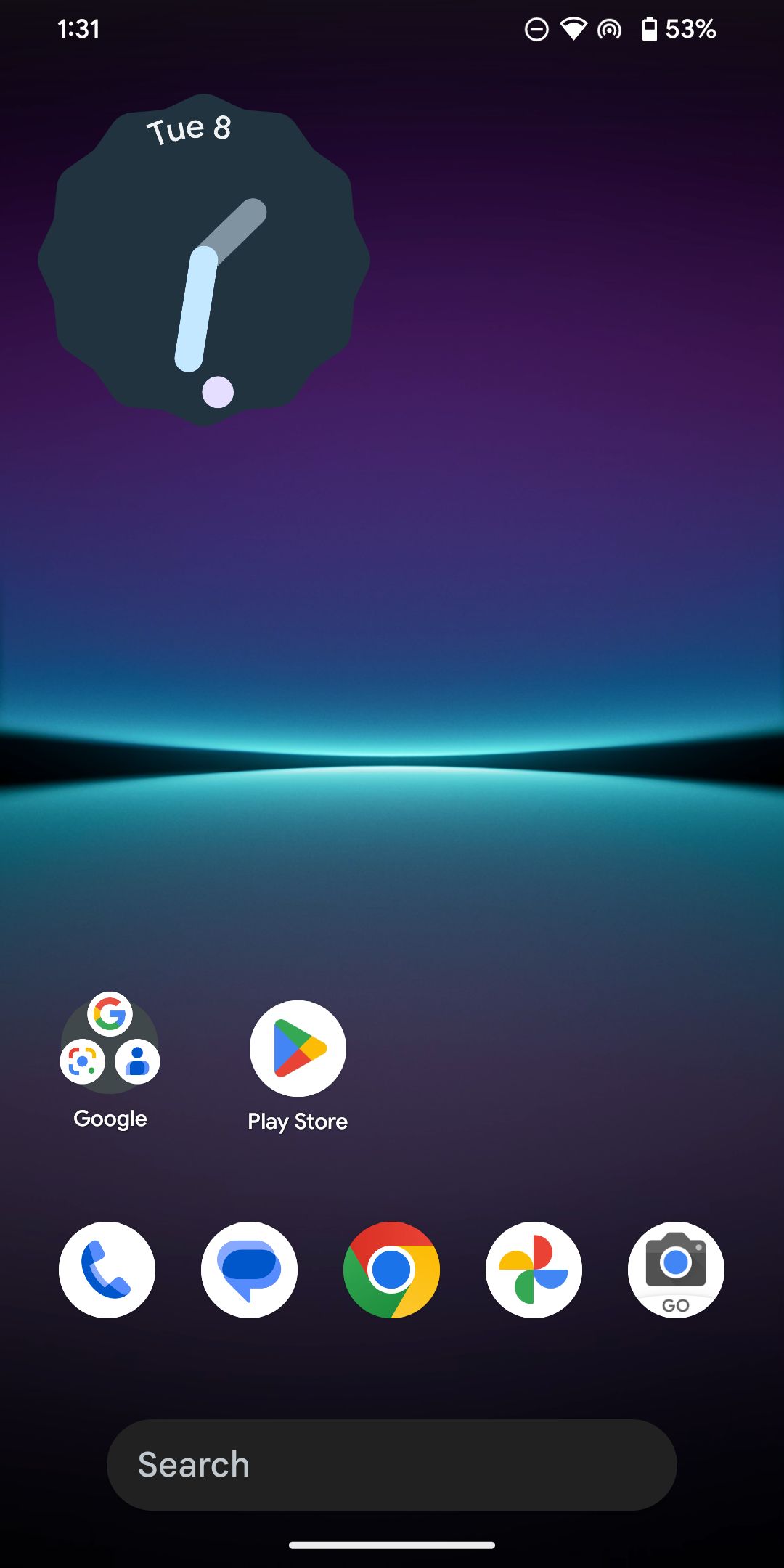The home screen depicted features a rich and vibrant color gradient background that transitions through various shades. Starting from the top, the background begins with black, moving to dark purple, then to purple, and progressively lightens into shades of teal, light bluish-green, back to black, and continues to white. This gradient then repeats in reverse with variations of light bluish-green, teal, light purple, and purple, eventually returning to black.

On the left-hand side, the screen displays the current time "1:31" in white text. Adjacent to this, there is a circle with a dash inside, indicating the "Do Not Disturb" mode. The Wi-Fi signal icon is also white, suggesting a strong connection. Beside it, a circle with lines indicates a possibly unknown function. The battery icon, also in white, displays "53%" charge remaining.

Towards the top of the screen, the date "TUE 8th" is prominently shown in uppercase letters along with an analog clock icon featuring blue and gray hands. Additionally, a very light pink circle can be found in this upper section.

At the bottom of the screen, there is a gray search box labeled "Search." Directly above this search box are five circular icons representing different applications: 
1. A blue phone icon.
2. A blue text box (possibly for messaging).
3. Google's "G" for the Google app.
4. Google Photos icon.
5. A black phone icon and a black camera icon, with the word "Go" underneath it.

This detailed description encapsulates the vibrant and organized layout of the home screen, highlighting its color schemes, functional icons, and app shortcuts.